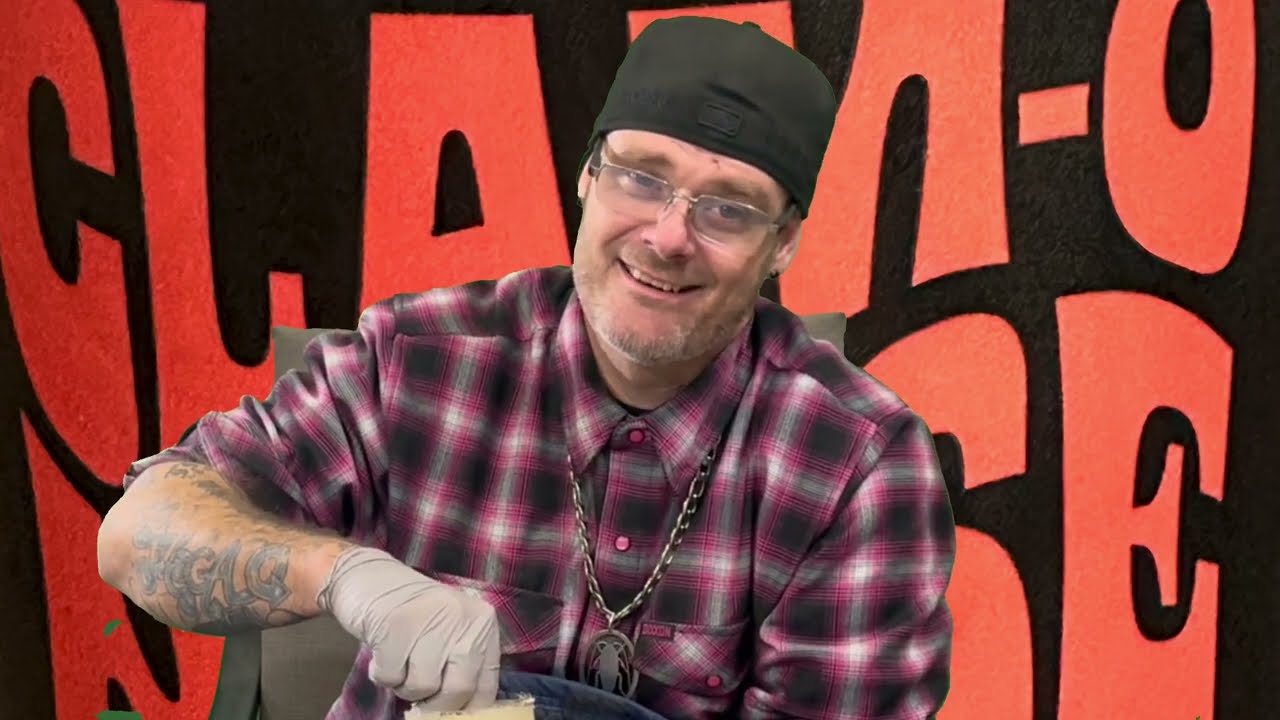The image showcases a middle-aged Caucasian man seated in a brown chair, smiling directly at the camera. He dons a black baseball cap turned backwards and wears clear-framed glasses. His light stubble beard, hinting at both gray and brown tones, gives him a rugged appearance. He is dressed in a plaid button-down shirt featuring red, black, and white colors, with the right sleeve rolled up to reveal a tattooed forearm. Around his neck hangs a thick silver chain adorned with a medallion that resembles a cockroach wearing sunglasses. Notably, his right hand, which is partially out of the frame, is clad in a gray rubber glove. Behind him, the black backdrop is strikingly adorned with giant all-caps letters in an orange bubble font, seemingly forming the partially obscured words "CLAM-O" and additional, unreadable text beneath it.